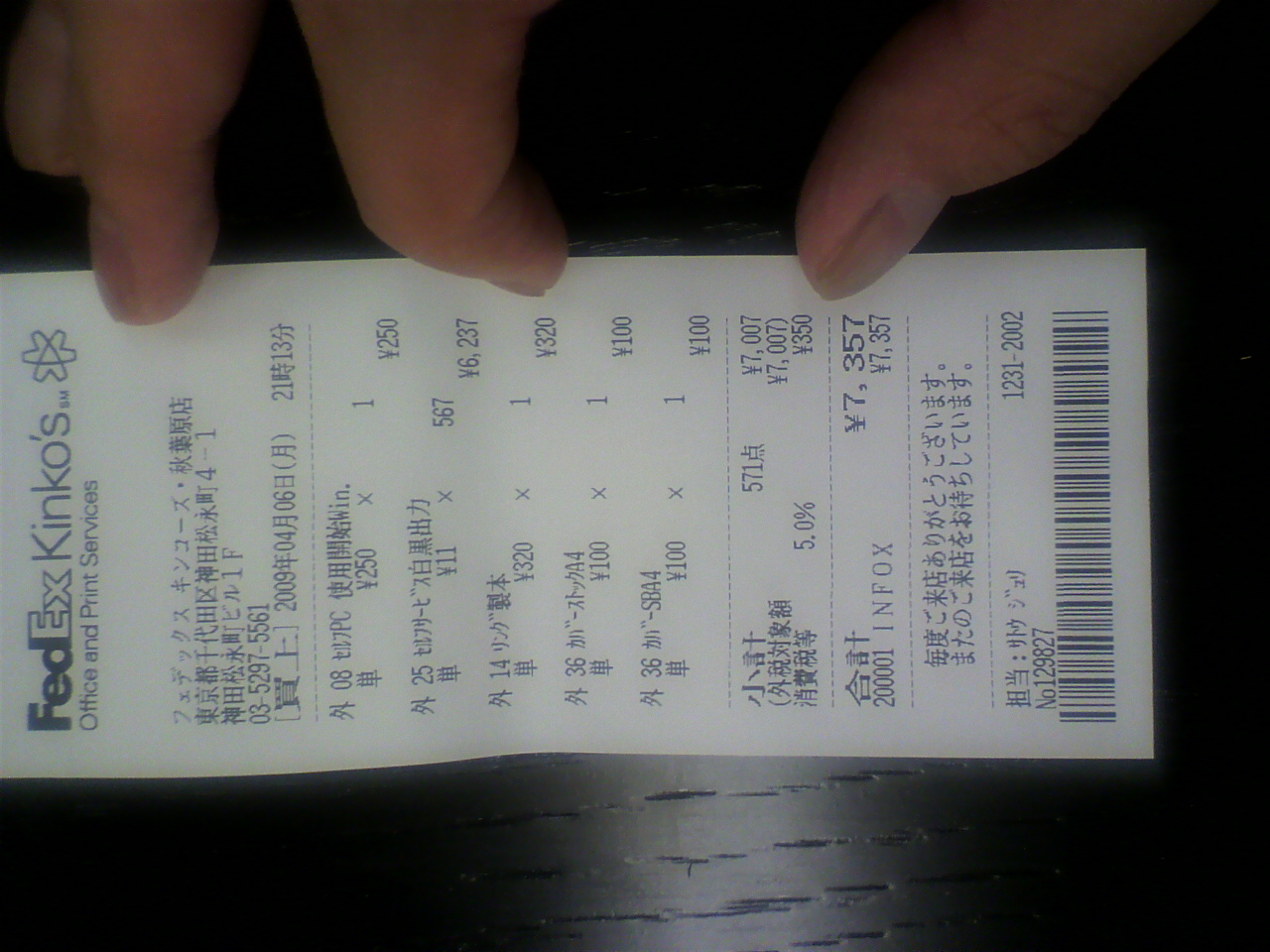This is a sideways photograph of a white FedEx Kinko's Office and Print Services receipt held down by a Caucasian person's hand, with their thumb, index finger, and forefinger visible, resting at the top edge of the receipt. The receipt appears to have been folded, and the hand is spreading it out on what looks like a dark, black-painted wooden surface. The photo quality makes it somewhat dark, but you can discern the wood grains. The receipt, written mostly in Japanese using kanji, katakana, and hiragana, displays various prices: 250 yen, 6,237 yen, 320 yen, 100 yen, and 100 yen, culminating in a total of 7,357 yen. Additional text on the receipt includes a contact number, 03-5297-5561, and 'InFox' near the bottom. The very bottom of the receipt contains a barcode for scanning.